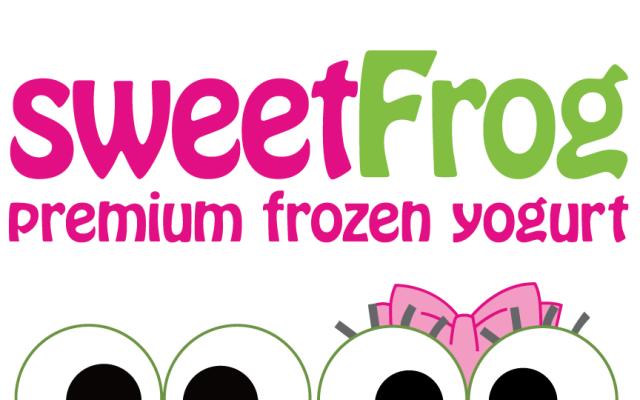The image depicts a simple yet vibrant logo for Sweet Frog Premium Frozen Yogurt set on a white background. Dominating the top third of the image is the text "Sweet Frog Premium Frozen Yogurt," with "Sweet," "Premium Frozen," and "Yogurt" in a bright pink font, while "Frog" stands out in a lighter green color. Below the text, in the bottom section, are two pairs of large cartoon eyes that give a playful and engaging feel. On the left, the eyes have a green outline with large black pupils, and on the right, a similar pair of eyes is adorned with a large pink bow and gray eyelashes, indicating a more feminine character. These elements—green frog eyes with a pink bow and a cohesive color palette of pink and green—combine to make a friendly and inviting logo that emphasizes the brand's fun and family-oriented atmosphere.